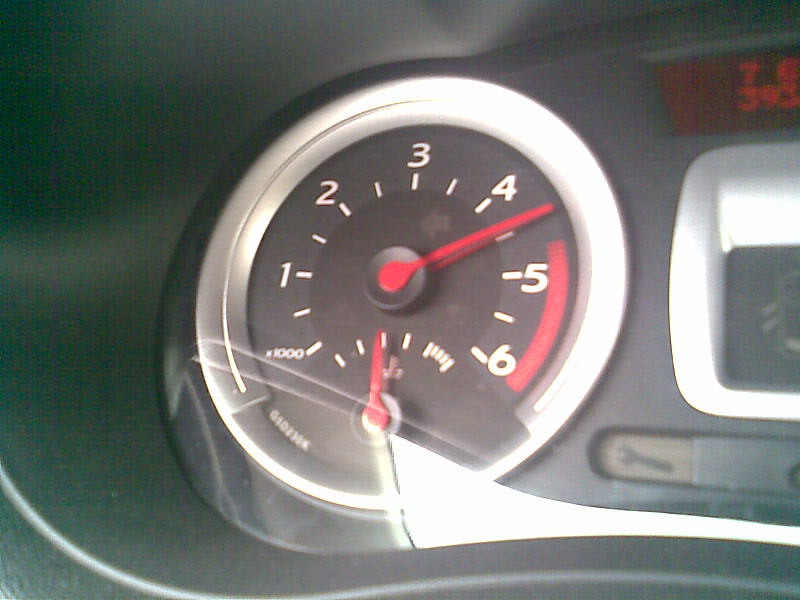This image showcases a detailed section of a car's dashboard, focusing primarily on the tachometer, which is prominently displayed in the center. The tachometer features red needles and is currently reading at 4.5 RPM. The tachometer is encircled by a sleek silver ring, and positioned immediately above it is a smaller gauge, also highlighted with red accents.

To the right of the tachometer, there is a digital display illuminated with the number "393," and near the top, there is another lit indicator. Adjacent to this setup, an element framed in white plastic can be seen, beneath which a warning light depicting a wrench is illuminated, signaling a required maintenance check or repair for the vehicle.

All the gauges, including the tachometer, are housed within a black plastic casing and are covered by a clear plastic shield for protection.